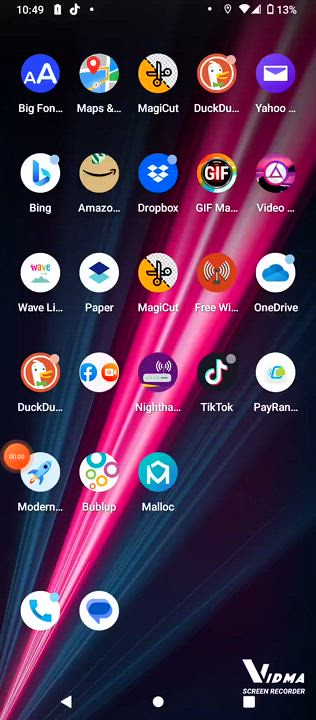This image is a detailed screenshot of a smartphone home screen. Displayed at the very top, the status bar shows critical information including the current time, Wi-Fi connectivity, battery level, and signal strength. A notable detail is the battery percentage, which is indicated as 13% remaining.

The layout of the apps follows a grid with five icons per row, each row showcasing a variety of applications. In the first row from the top, the apps listed are BigFont, Maps, Magic Cut, DuckDuckGo, and Yahoo. The second row features Bing, Amazon, Dropbox, GIF Maker, and an app labeled 'Video,' although some app names are partially cut off. Moving down to the third row, the displayed apps are Wave, an app with 'Light' in its name, Paper, Magic Cut, and Wi-Fi Free, along with OneDrive. The fourth row includes DuckDuckGo, a folder labeled 'Group of Apps,' Nighthawk, TikTok, and an app labeled PayRan.

At the bottom of the screen, a fixed dock contains essential communication apps—Phone and Text.